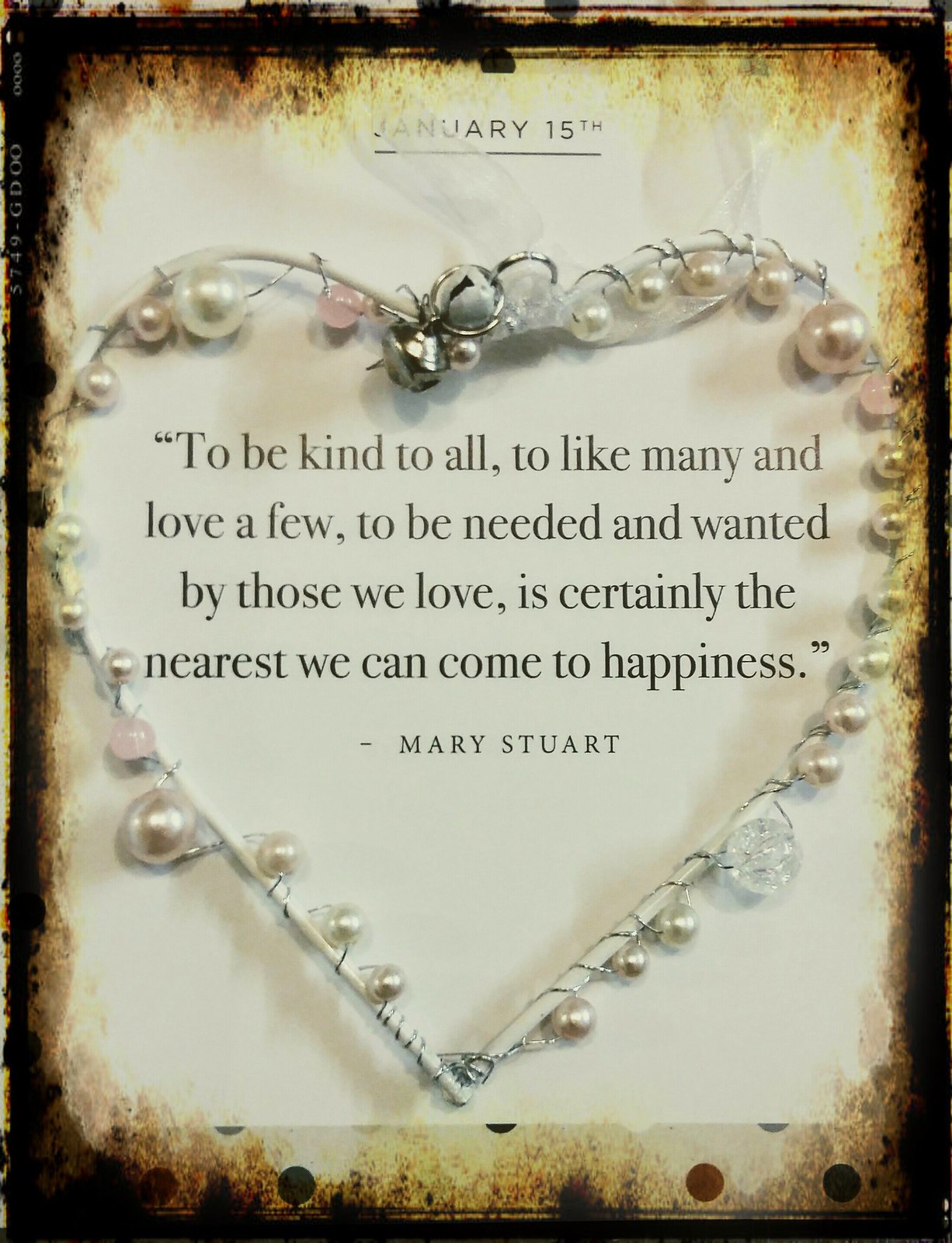The background of the image resembles a piece of old, worn parchment paper, with burnt and soot-stained edges. Centered on the paper is a wire sculpture in the shape of a heart, entwined with strands of metal wire adorned with an array of beads and pearls, including some crystal elements. At the top center of the heart, there is a small, delicate bell. Above this heart, the date "January 15th" is prominently displayed. Underneath it, in the middle of the image, a beautifully penned quote reads: "To be kind to all, to like many and love a few, to be needed and wanted by those we love, is certainly the nearest we can come to happiness." This quote is attributed to Mary Stewart, with her name appearing below it. The overall aesthetic suggests an inspirational or sentimental feel, enhanced by the intricate details of the heart ornament and the profound simplicity of the quoted words.